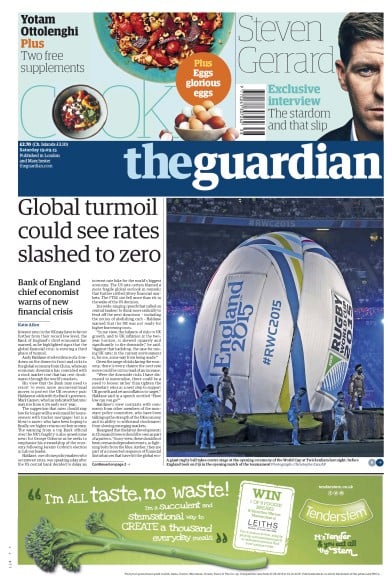This image portrays a newspaper with multiple headlines and vibrant colors. Prominently featured in the upper section is the headline: "Bank of England Chief Economist Warns of New Financial Crisis." Accompanying this segment, subheadlines read: "Stephen Girard, Exclusive Interview," "This Tardown and That Slip," and "Global Turmoil Could See Rate Slashed to Zero." To the right, the paper highlights the "England 2015 Rugby Cup" with an image of a stadium packed with an enthusiastic crowd. 

Towards the lower part of the page, several advertisements are visible. One promotes a product with the catchy lines: "An Old Taste, No Waste," and "A Succulent and Stem-sational Way to Create a Thousand Everyday Meals," featuring the slogan, "Tender Stem — It's Tender and You Eat All the Stem."

The overall palette of the image is rich with hues of orange, red, blue, white, black, and green, creating a striking and visually appealing presentation.